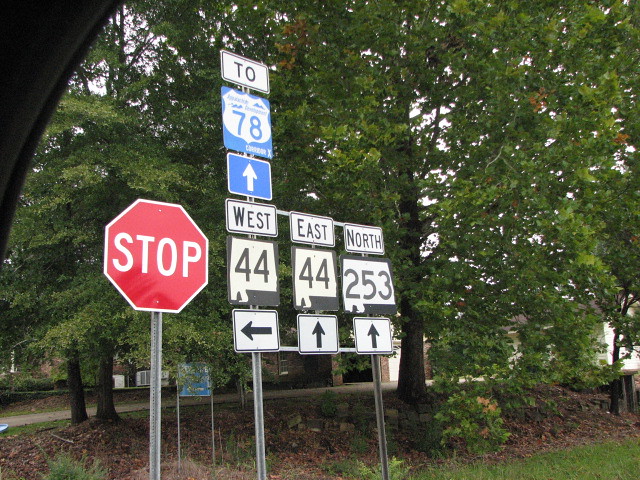This photograph captures a close-up of a cluster of road signs situated along the side of a road, positioned amid a grassy area. Behind the signs, a dense collection of tall trees, adorned with full green leaves, provide a verdant backdrop. Nestled behind these trees is what appears to be a walking path, leading to the red brick exterior of a building featuring a white garage door, possibly indicating a residential driveway.

The road signs are arrayed on a metal frame that rises vertically, extends horizontally, and then descends on the other side, holding nearly 10 different signs. Closest to the road stands an outermost stop sign. Adjacent to it are several directional and route signs: a leftward arrow, two straight-ahead arrows, West 44, East 44, and North 253 route markers. Above these, a small blue square sign with a white border and a white arrow points straight ahead. Near the top of the frame is a State Route 78 sign, while crowning the display is a small rectangular sign bordered in black that reads '2' in black letters.